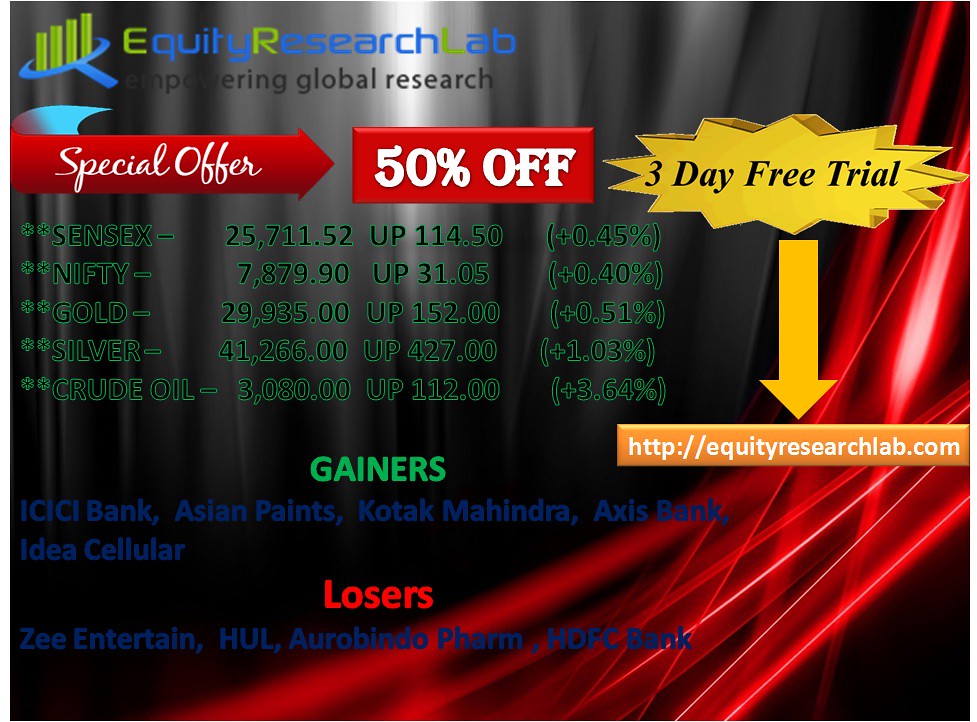The image is a screenshot of an advertisement for the Equity Research Lab, prominently featuring a gray and white background with a red stripe along the right side. At the top, "Equity Research Lab" is written with the first letter of each word in green and the remaining letters in blue. Below this, "Empowering Global Research" is displayed in black text. A red arrow pointing to the right contains the words "Special Offer" and leads to a red box with white lettering stating "50% Off." Adjacent to this box is a starburst icon with the text "3-Day Free Trial." A yellow arrow below points downward to the website, equityresearchlab.com.

Underneath the offer section, there is financial information on various assets. To the left, it lists Sensix, NIFTY, Gold, Silver, and Crude Oil, showing their current values and percentage gains in green. Specific numbers indicate updates, such as Sensix at $25,700.52, up by $114.50 or 0.45%. Below this financial data, there is a breakdown of gainers and losers. The gainers, listed in green, include ICICI Bank, Asian Paints, Kotak Mahindra, Access Bank, and Idea Cellular. The losers, written in red, feature Z Entertain, Hull, Aerobindo, Farm, and HDFC Bank. The layout of the advertisement is well-spaced with no central focus, aiming to direct viewers to their website for more details on their financial services.